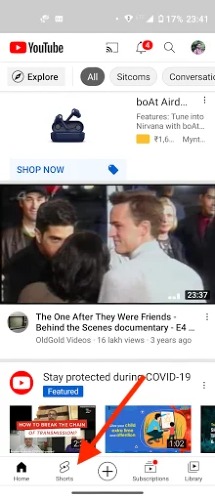Caption: 

The image features a busy scene reminiscent of a behind-the-scenes documentary, highlighting various elements of modern life and media. In the foreground, there's a person in a white suit interacting with another individual wearing a blue shirt and black pants. They appear to be engrossed in a conversation, possibly discussing a popular sitcom titled "The One After," which prominently features themes of friendship. Various notifications and icons pepper the surroundings, including a red dot indicating four new notifications and a globe icon.

The backdrop includes visual cues that hint at a production or technology-related environment: a TV screen displaying "The One After," and various labels like "Stay Protected," likely a nod to COVID-19 precautions. There's also a "Shop Now" button with a blue tag promoting Bluetooth headphones and Wi-Fi connectivity, suggesting a campaign for these products.

Additionally, a banner displaying "17% Subscriptions, Explore, and Library" points towards a streaming service or platform, while the presence of icons like a cast button and three vertical dots signifies a menu for further options. The numbers 2337, 2341, and 102 could be reference codes or viewer counts, with the mention of "Views, Three Years Ago, Number 1.6 LAKH" specifically referring to the popularity and timeline of an "Old Gold Video" or possibly a song from Nirvana with Boat.

Overall, the caption paints a picture of a vibrant blend of media consumption, technology, and promotions set against the backdrop of a bustling, modern information age.